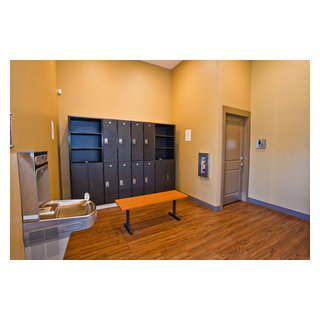The photograph depicts a small, likely gym locker room characterized by its beige walls and an orange-toned wooden floor. Dominating the back wall are two levels of black or gray lockers; the upper row features shelves on either side with three compartments each, while the lower row consists entirely of lockers extending to the floor. A wooden table with black legs stands in front of these lockers. To the left side of the image, a stainless steel drinking fountain is mounted on the wall, which also includes an alcove. On the right side, a beige door, possibly with a sign to its right, is partially visible. The room appears empty, with no sports equipment or people present, and has an apricot-colored ceiling. The overall scene conveys a sense of vacancy and potential, leaving the function and current use of the space open to interpretation.